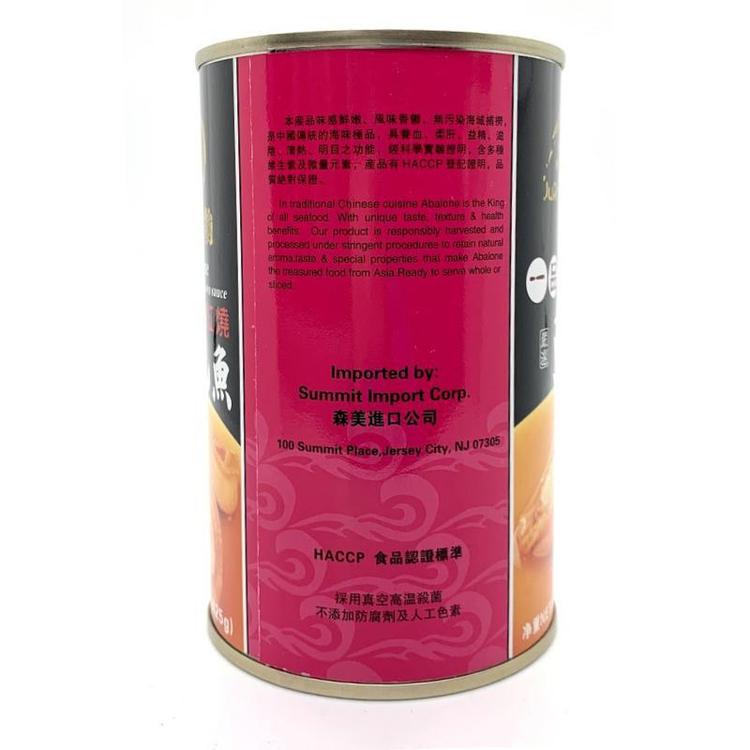This image features a large, somewhat older-looking steel can set against a solid white background. The can is predominantly pink, with additional hues of dark pinkish-red, black, and beige dispersed throughout. The focal point of the can includes various oriental characters, specifically Chinese text, suggesting it contains a product used in traditional Chinese cuisine. The can further includes English text indicating it was imported by Summit Import Group situated at 100 Summit Place, Jersey City, New Jersey, with additional mentions of HACCP certification. The can's design includes silver lips on the top and bottom edges, with the pink section being the most dominant color. The detailed English description highlights the product's unique taste, texture, and health benefits, and mentions that it is ready to serve whole or sliced.